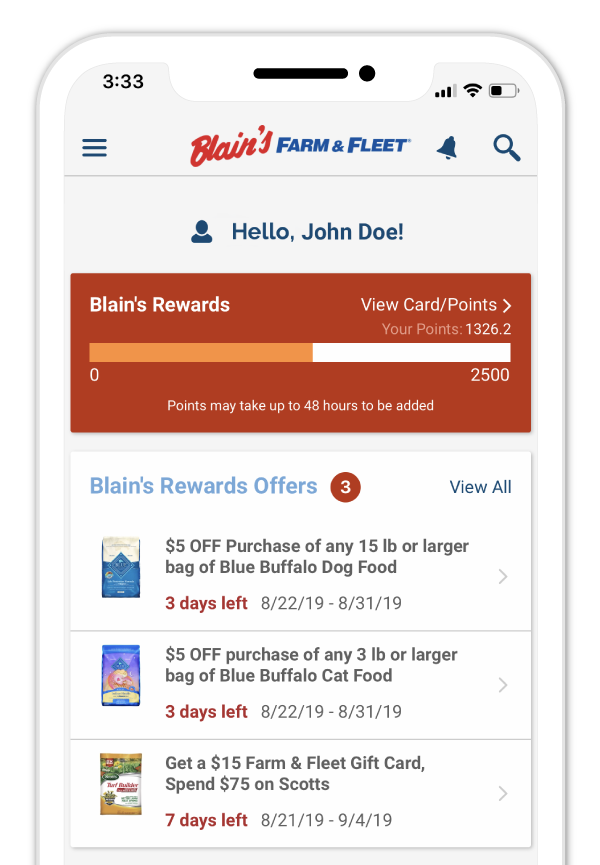The screenshot features a smartphone displaying the Blair's Farm and Fleet website, where the user is logged into their account. The phone's outline is gray, and the screen background is white. At the top left corner, the time is displayed as 3:33, and on the top right, there are three out of four bars indicating signal strength. The phone is connected to Wi-Fi, and the battery is half full.

Below the status bar, the navigation area includes three horizontal black lines on the left, the site name "Blair's" written in italic red font, followed by "Farm and Fleet" in bold blue. To the right, there’s a notification bell and a magnifying glass icon.

Beneath this, a gray line appears with an icon of a head and shoulders next to the greeting "Hello, John Doe." Below this greeting, a red bar indicates the user's reward status with Blair's. The top section reads "Blaine's Rewards," with the text "View Card Points" and "Your Points 1326.2" beneath it. An orange and white bar graph shows points ranging from 0 to 2,500, with a caption stating that "Points may take up to 48 hours to be added."

The webpage lists three available offers, highlighted by a red circle with the number three. The first offer features a bag of Blue Buffalo dog food, colored white and blue, with a discount of $5 off on any 15-pound or larger bag. The offer period is displayed in red font, running from 8/22/19 to 8/31/19, with a three-day countdown.

The second offer is for Blue Buffalo cat food, depicted in a blue bag with a tan puppy on it. This deal also offers $5 off, but for any three-pound or larger bag, with the same validity period from 8/22/19 to 8/31/19, and three days left.

Finally, there's an offer for a bag of Scott's lawn treatment, which comes in a white bag with yellow and green graphics. The deal includes a $15 Farm and Fleet gift card upon spending $75 on Scott's products. This offer spans from 8/21/19 to 9/4/19, with seven days remaining. Each offer has a right-facing caret on its right-hand side for more information.